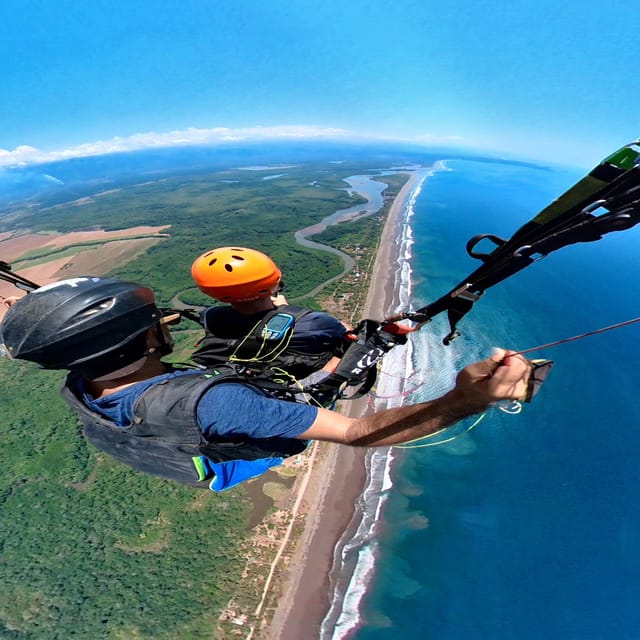This captivating fisheye lens photo captures a breathtaking aerial view of two skydivers in tandem, floating high above a scenic coastal landscape. The individual in front is wearing an orange helmet, while the person behind, possibly the instructor, dons a black helmet and a blue shirt. The instructor is gripping a red cord, indicative of the parachute being deployed. The coast sprawls beneath them with a sandy beach stretching along the bottom of the image, bordered by the ocean to the right, where white waves crash against the shore. To the left, lush green foliage dominates the terrain, punctuated by a small river flowing towards the ocean. A dirt road can also be glimpsed winding through the greenery. The sky is a vivid blue, adorned with a few scattered clouds, and the curvature of the horizon is subtly curved due to the lens, offering a surreal and expansive view of the island they're soaring over.